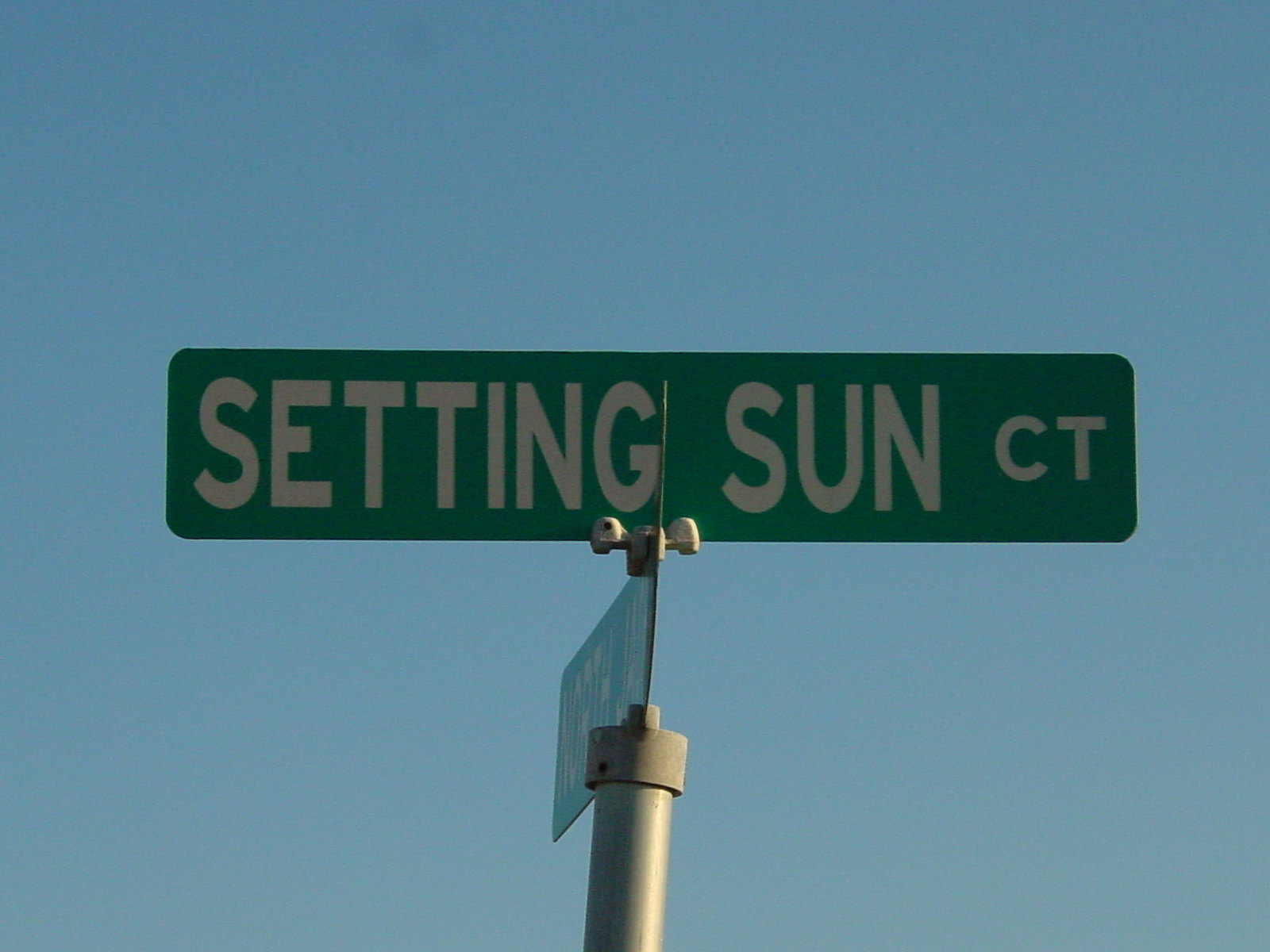The image depicts a street sign at an intersection during dusk, where the sky is a clear blue and the sun is setting. The photograph is taken from a slightly low angle, looking up at the sign. The main sign, which spans left to right, reads "SETTING SUN CT" in all capital letters and is mounted on a gray metallic pole. A second, smaller and less readable, green sign seems to indicate "North" perpendicular to the main sign. The street signs are new and feature an attractive font. Sunlight illuminates one side of the pole, highlighting the simple, reflective design of the street signs against the serene backdrop of the evening sky.